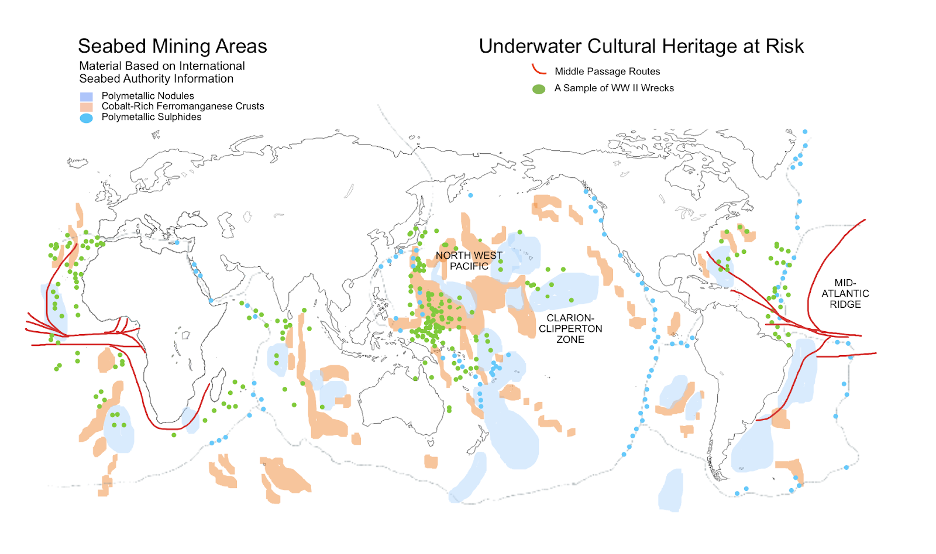This detailed map, based on information from the International Seabed Authority, illustrates various seabed mining areas and underwater cultural heritage at risk. On the top left corner, labeled in black, it reads "Seabed Mining Areas," and includes a legend with a purple rectangle indicating polymetallic nodules, a peach rectangle for cobalt-rich ferromanganese crusts, and a blue oval denoting polymetallic sulfides. On the top right, labeled "Underwater Cultural Heritage at Risk," it features a red line representing middle passage routes and green circles that signify World War II wreck sites. The central part of the map includes notable regions such as the Northwest Pacific, the Clarion-Clipperton Zone, and the Mid-Atlantic Ridge, marked with various colored dots and lines highlighting key areas and interests. Africa is positioned on the right, with North and South America on the left, and Asia in the middle, enhancing the geographical context of these critical seabed locations.